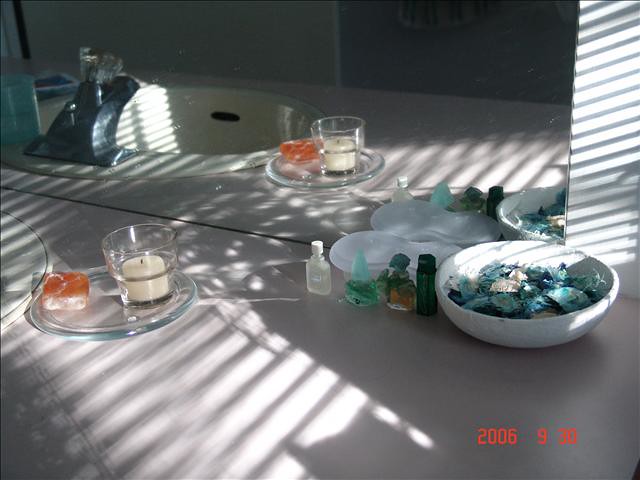This image, captured indoors, likely in a bathroom, dates back to September 30th, 2006, as noted by the timestamp "2006 930" in the bottom right corner. The scene features a light-colored Formica countertop extending across the lower portion of the photo, adorned with various bathroom items. To the right, the counter is bathed in a pattern of light and shadow cast by Venetian blinds, their slats distinctly outlined against the surface.

Dominating the scene is a large mirror, reflecting the sink area. The sink, positioned centrally, is equipped with a single crystal plastic faucet knob and features a visible drain outlet at the front. Notably, an aqua-colored accessory, possibly a soap dispenser, and a towel rest to the left of the faucet in the reflected view.

Focusing back on the direct image, just above the sink's outline, there is a soap dish with a reddish-amber bar of soap and a white crystal glass containing a small white candle. At the base of the mirror, in the lower right, four perfume bottles are neatly arranged: a white bottle, a green bottle with a bluish cap, an amber bottle with a pewter cap, and a black bottle. Near these is a creamy white object, resembling the shape of a shoe, though its exact function is unclear. Adjacent to this is a ceramic white bowl brimming with potpourri, featuring a mix of blue, white, and green petals.

The reflection in the mirror extends to show part of the bathroom wall—darker on the right and lighter with a white strip on the left. The upper left corner of the image showcases alternating dark and white strips, hinting at the possible presence of a closet door.

This detailed depiction captures the serene and organized setting of a 2006 bathroom, highlighting both its practical elements and touches of personal style.